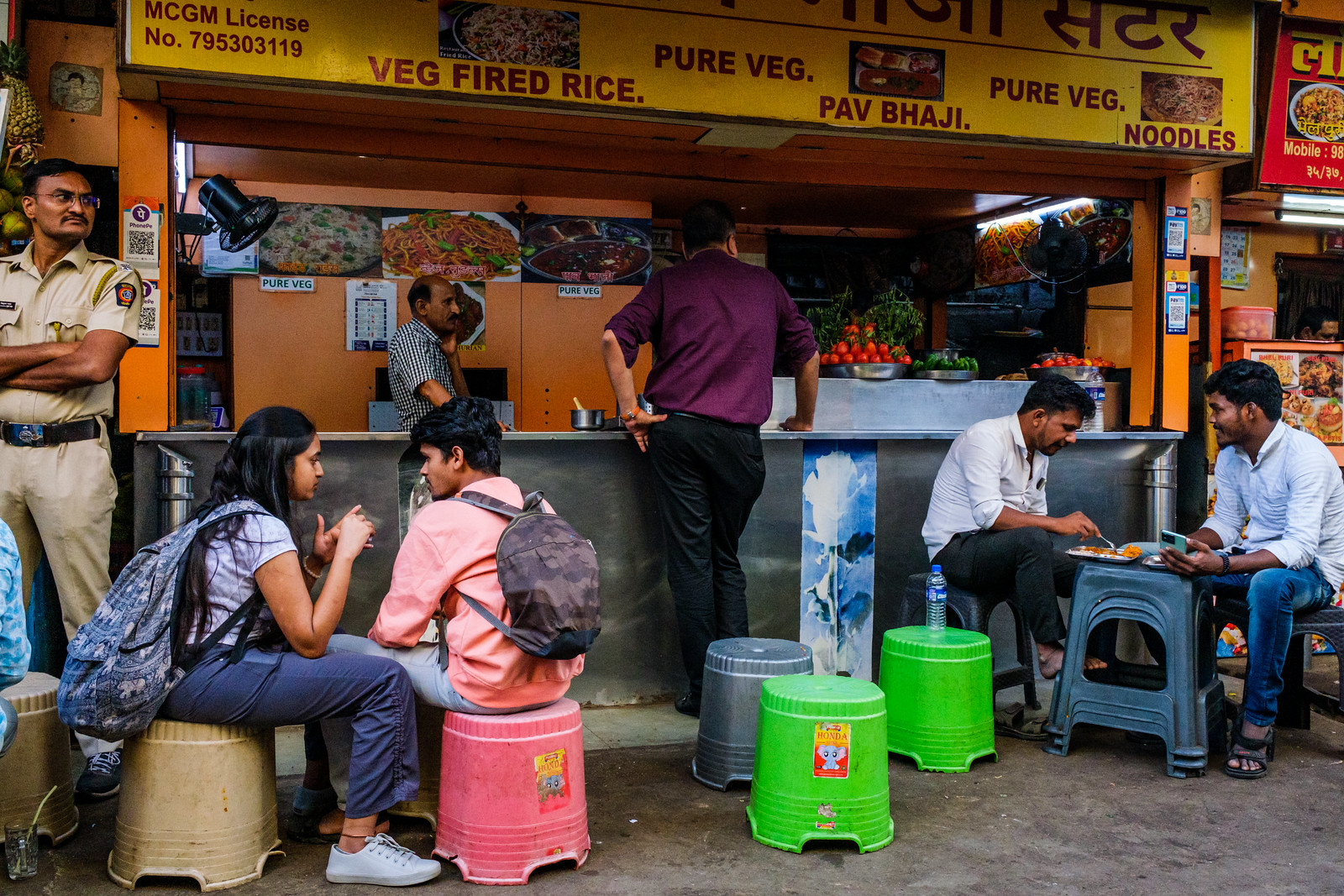The photograph captures a vibrant scene outside a food stall with a cropped banner featuring a yellow background and dark red text listing items such as veggie fried rice, pure vegetable dishes, pav bhaji, and noodles. Various images of these food items are also displayed. Four people are seated on little plastic stools and upturned buckets, engaging in conversations and eating. Among them are two younger individuals with backpacks sitting closely together on the left. A small plastic table with more gray-green buckets is situated in the middle where two men are eating, one looking down at his food while the other gazes across the table. To the right, fresh vegetables like tomatoes can be seen in small bowls. Two men are attending the counter: one wearing a purple shirt standing in front and another in a black and white checkered dress shirt behind the counter, glancing to his right. To the left stands a guard in a beige outfit with arms folded, watchfully overseeing the bustling scene. Another stall is visible at the right edge of the image, completing the lively market atmosphere.